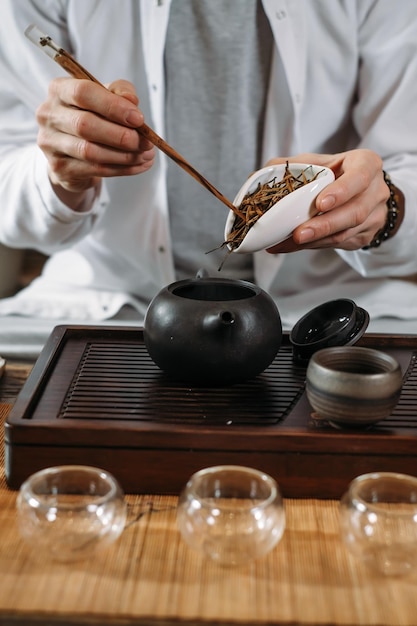In this image, we see a person, presumably a scientist or meticulous artisan, engaged in what seems to be a precise, detailed experiment or preparation ritual. The individual, dressed in a white lab coat or light-colored attire layered over a gray shirt, is partially visible from the chest up, emphasizing a focus on the task at hand. They are using a long, brown tweezer-like utensil in their right hand to delicately extract and guide a collection of brown, grassy sticks, potentially dried tea leaves, from a small, white, cup-like container in their left hand. This substance is being carefully transferred into a small, dark gray (almost black) teapot situated on a brown wooden surface with horizontal slits, possibly serving as a makeshift heating pad or surface with a rustic aesthetic. The teapot's spout is directed towards the viewer, suggesting an invitation to observe the process. To the right of the teapot, there is its lid lying on its side and another small silver pot beside it. In the foreground, three clear glass bowls rest on the same brown wooden surface, adding to the image’s meticulous and organized composition.